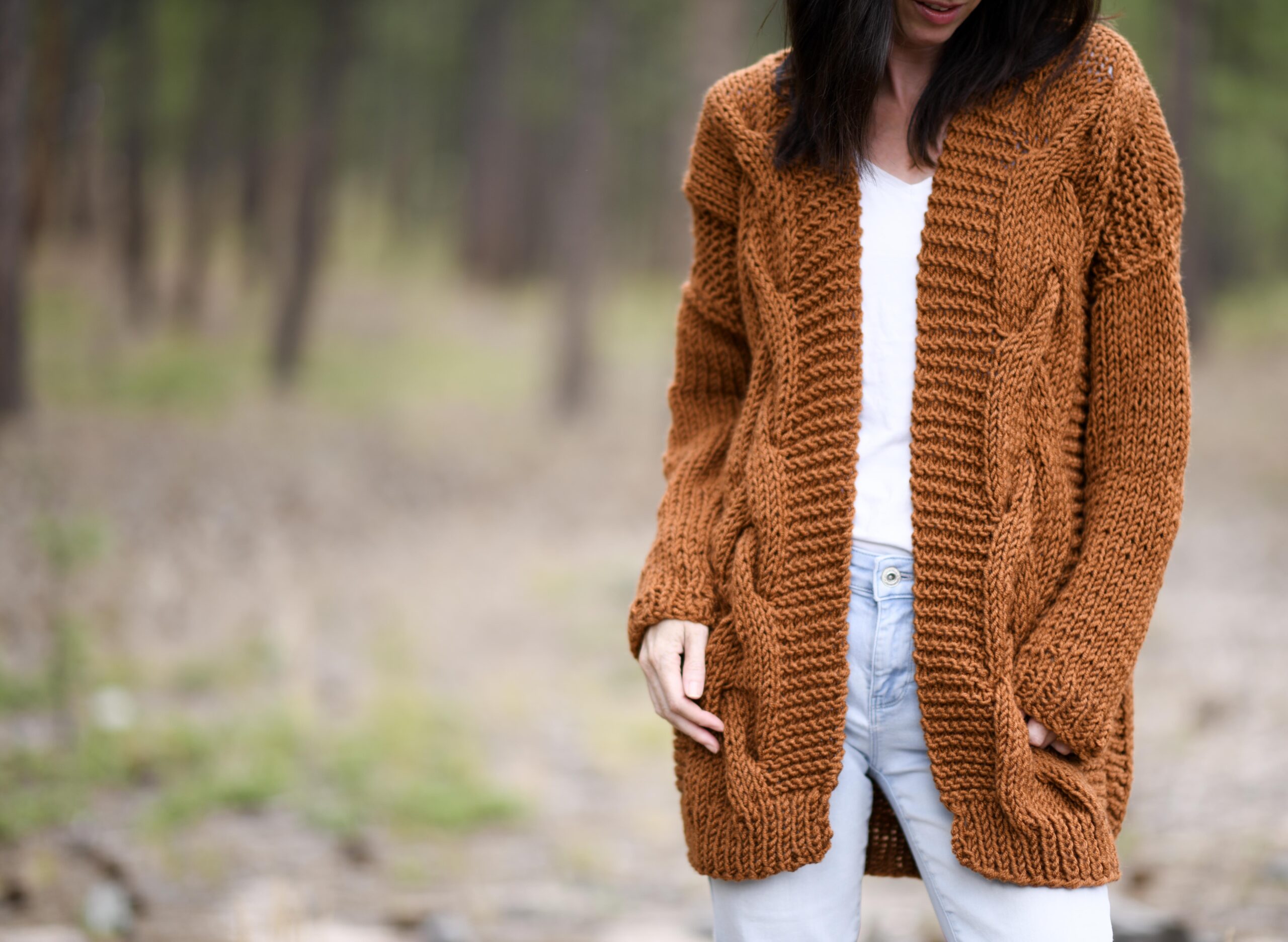This is a photograph of a young woman, likely in her twenties, standing outdoors in what appears to be a wooded area. Captured from just below her mouth down to just above her knees, the focus of the image is the woman's clothing and the background, which is significantly blurred. She has long, dark brown, almost black hair that cascades over her shoulders down to her chest, and she seems to be smiling. She is dressed in a traditional, elaborately cable-knit brown sweater, which is open at the front and extends over her hips, with sleeves that partially cover her hands. Underneath, she is wearing a white top paired with light blue, slightly faded jeans. The background, while extremely blurry, hints at a sparsely wooded area with predominantly brown tones and hints of green grass on the ground, contributing to the overall natural and serene setting of the photograph.